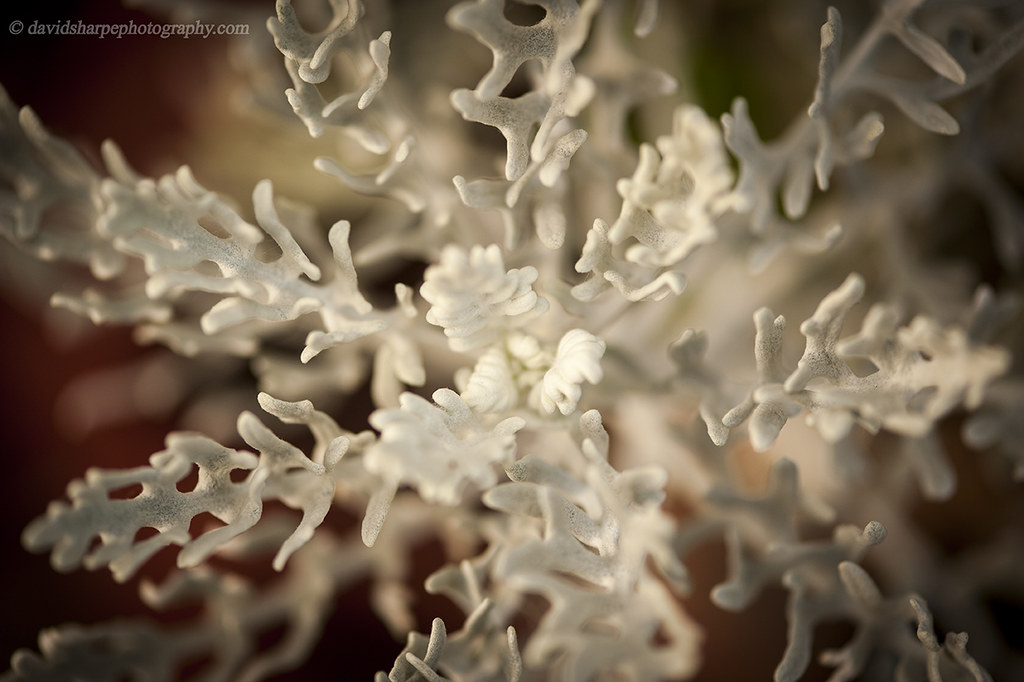This is a detailed, top-down photograph of an intriguing white object that appears either like dried leaves, a unique flowering plant, or possibly coral. The primary focus is on the main structure, which is centrally positioned and composed of numerous branches or stems. These branches fan outward from the center, giving it an organic snowflake-like appearance. The white material has an almost plastic, fuzzy, or sandy texture. Out-of-focus branches and stems with similar white spikes are visible in the background, enhancing the depth of the image. The background itself transitions from black to red towards the center. At the top left corner, there is a small text that says "copyright davidsharpphotography.com". This captivating photograph manages to blend the details of natural and potentially artificial elements in a visually striking manner.